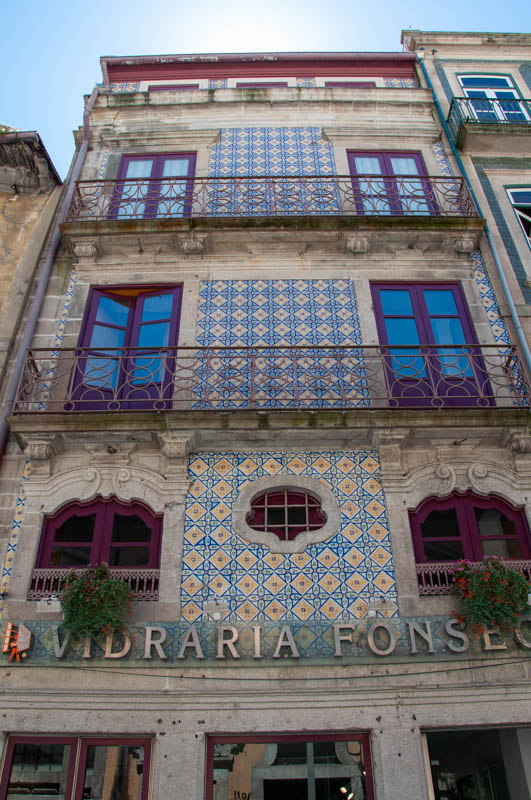The image captures the front of a multi-story building named Vidraria Fonseca, which appears to be a hotel with architectural influences that hint at Middle Eastern or possibly Cuban designs, reminiscent of an old Arabian city or Miami themes. The perspective is from the street, looking up at a sharp angle. The building has five distinct levels, though the bottom is partially cut off, revealing only the tops of probable windows and an entrance door to the left. 

The facade prominently features text reading "Vidraria Fonseca," situated above a tiled wall adorned with a blue and yellow pattern. Red window shutters with lush flowers underneath add a splash of color to each level. The second and third levels each boast narrow balconies with railings and purplish-colored doors on either side. These doors likely lead to the hotel rooms, which consist of two rooms per level, adding up to six rooms in total. Both stories above mirror this layout, while the topmost tier culminates in a red roof. On either side of the main hotel name, there's an associated image. The clear daytime sky indicates that the photograph was taken in bright sunlight, enhancing the vividness of the building’s colorful details.